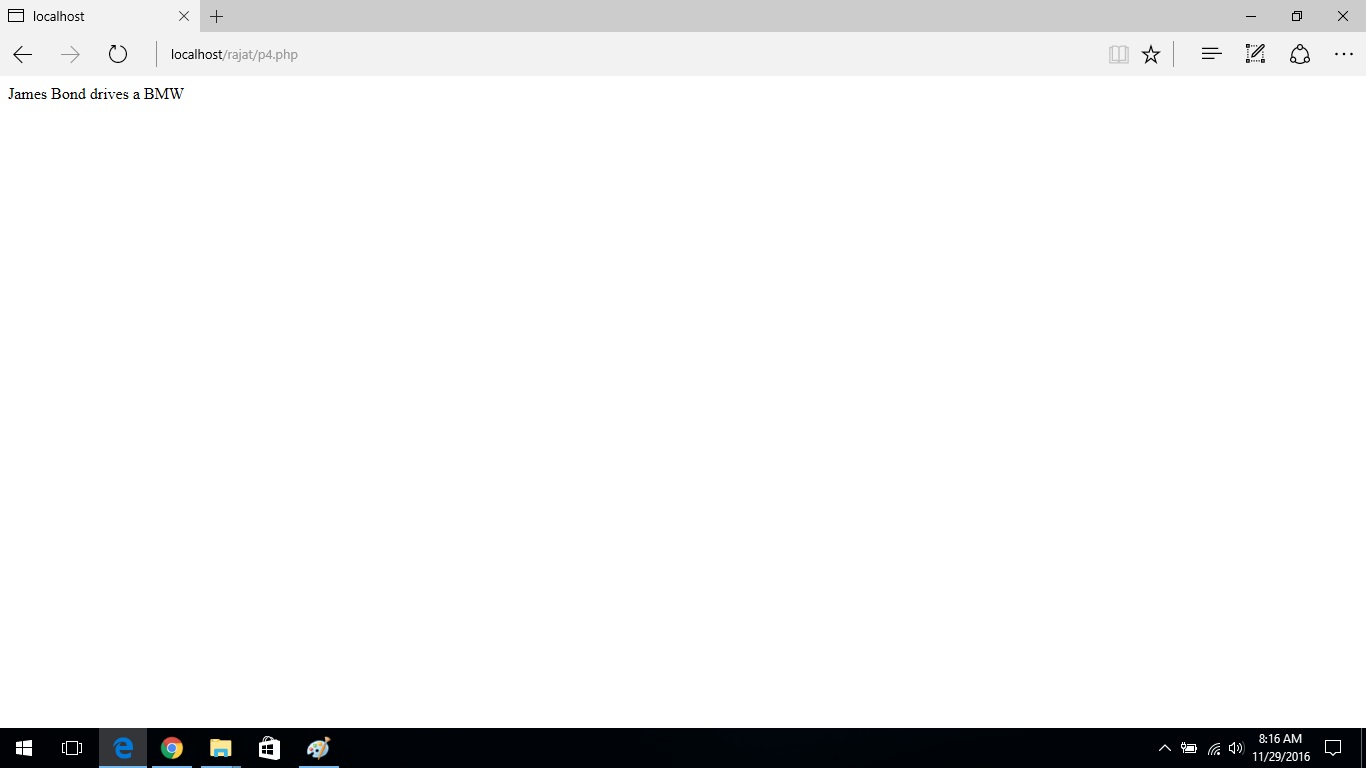A screenshot of a webpage is depicted in the image. The central portion of the screen is entirely blank, featuring only a white background. At the top, the browser's standard toolbar is visible, showing a single open tab with a plus sign beside it for adding a new tab. The top-right corner of the browser contains the usual window control buttons: an expand icon and an 'X' to close the page.

In the light gray navigation bar, there are left and right arrows for page navigation, and a refresh button. The URL displayed in the address bar reads "localhost/p4.php." To the right of the address bar, there are icons for bookmarking (a star), text justification options, editing, and a menu represented by three vertical dots.

Below the address bar, in the top-left corner of the white space, the text "James Bond drives a BMW" is prominently displayed. The rest of the white space remains empty.

The bottom portion of the screenshot displays the Windows taskbar, featuring the Start menu icon, shortcuts to Internet Explorer, Mozilla Firefox, File Explorer, Paint, and other applications. The system tray at the bottom-right corner shows the date and time, along with other system indicators.